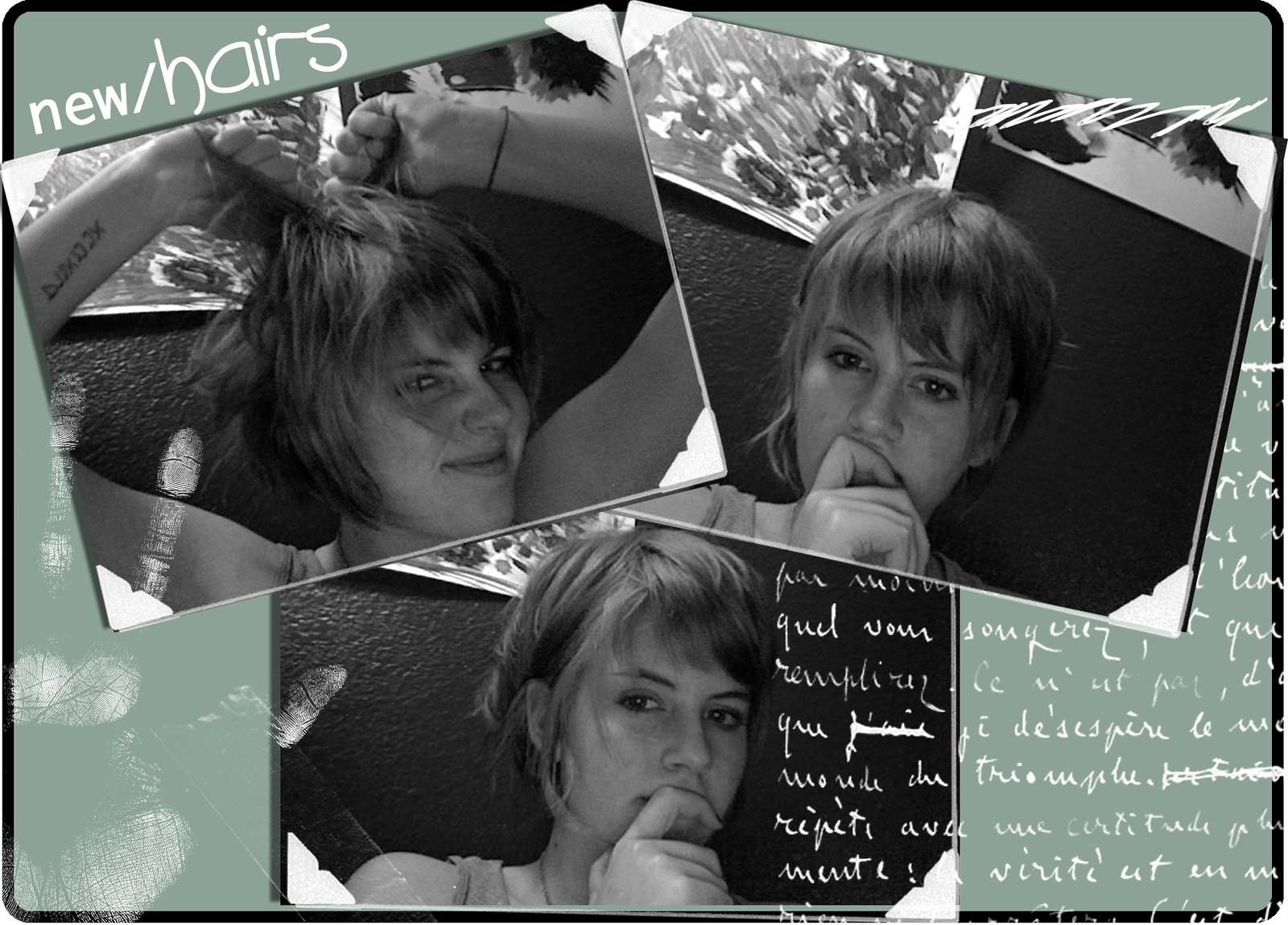This image is a collage of three black-and-white photos of the same woman showcasing different hairstyles and expressions. The main frame has a black border, and the background is a soft olive green with handprints and fingerprints scattered across it. At the top left corner, there is a caption that reads "New Hairs" in large, mixed-case letters. 

In the first photo, located at the top left, the woman is pulling her short chin-length hair upward with both hands. She is wearing a sleeveless shirt and looking to the side, with a tattoo visible on her right forearm. Adjacent to this, on the top right, is another photo of the same woman, this time with her finger resting on her lips, appearing to be in deep thought. She is wearing a tank top, and her hair, still short at chin length, looks more organized and not frizzy.

The final picture at the bottom center also features the woman with her finger on her lips in a similar contemplative pose but looking in a different direction. All three photos have a consistent black background, and the middle and bottom photos contain some cursive handwriting that is difficult to read. Additionally, there are words such as "far," "move," "quill," and "defy" visible beside the bottom photo. The right side of the collage has more handwriting in another language, likely cursive, on a green background.